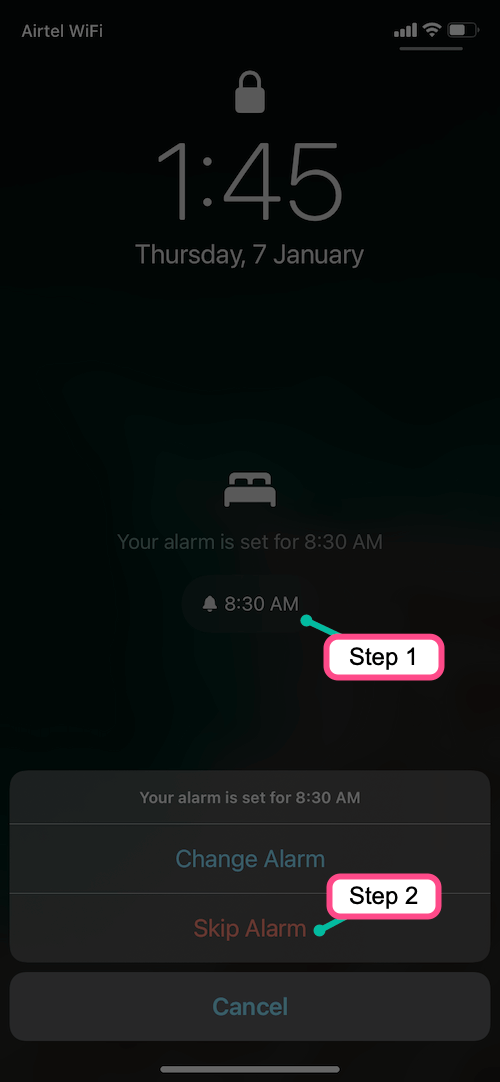The image depicts a screenshot from a cell phone. The background is a vertically oriented black rectangle. In the upper left corner, the text "Airtel" is displayed in gray, alongside the term "Wi-Fi". To the right of this text, the signal strength is shown with full bars, and the nearly full battery icon is colored light gray. Additionally, there is a lock symbol indicating the phone is secure. Directly below these icons, the time is displayed as 1:45 PM, followed by the date "Thursday, 7 January".

Approximately three inches down from the top of the screenshot, there is an icon resembling a bed, represented as a long rectangle with two small squares on top. Next to this icon is a message stating, "Your alarm is set for 8:30 AM," accompanied by a gray bell icon and the text "8:30 AM". A green line extends from the "AM" and connects to a pink square. Inside this pink square, the text "Step 1" is written in black over a white background.

Further down the screen, near the bottom, there is another pink square marked "Step 2", connected by a green line. Inside this square, the text "Skip Alarm" is displayed in pink. Below this, the word "Cancel" is written in blue text, and above it, another blue text states "Change Alarm".